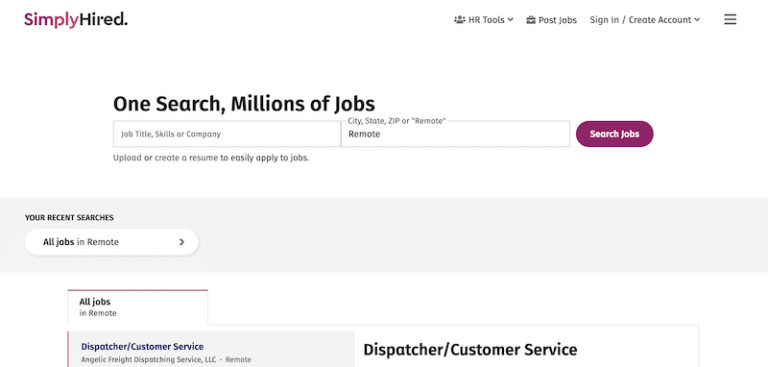The image is a horizontal screenshot of the Simply Hired website, with a clean, white background seamlessly blending with the screen’s whitespace.

In the upper left corner, the Simply Hired logo is prominently displayed. Moving right across the top navigation bar, there are several options: 'HR Tools,' 'Post Jobs,' 'Sign In / Create Account,' and an icon with three horizontal lines indicating a menu for additional options.

A headline in bold black text towards the left reads, "OneSearch, millions of jobs." Directly below are two search boxes: one to enter a job title, skills, or company, and the other for city, state, zip, or remote jobs. Adjacent to these boxes is a purple button labeled "Search Jobs" in white text.

Below the search functionality, a prompt encourages users to "upload or create a resume to easily apply to jobs," followed by a gray box containing information about recent searches. In bold black text, it states "Your recent searches," and lists "All jobs in remote."

Further down, within another gray box, there is a specific job listing highlighted in blue text: "Dispatcher / Customer Service, Angelic Freight Dispatching Services, LLC - Remote." To the right, in a white box with bold black text, the job title "Dispatcher / Customer Service" is repeated.